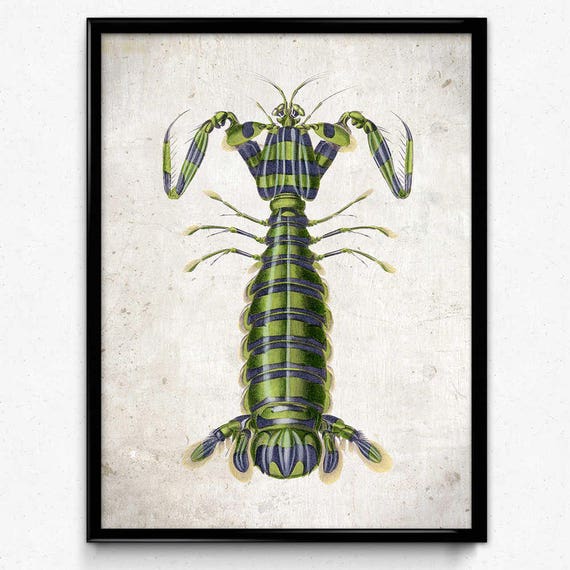This image features a whimsical, framed painting of an insect that blends imaginative elements with realistic details. The insect, depicted on a faded ivory or speckled dirty white canvas, is enclosed in a black frame hanging on a wall. It appears to be a fantastical hybrid, merging characteristics of a praying mantis and a beetle. The insect exhibits a long, green body adorned with purple and blue horizontal stripes. Its unique anatomy includes two large claw-like appendages emerging from its shoulders, two smaller arms pointed towards its chest, and six segmented legs—three on each side—attached to its upper body. The insect's head is positioned forward, crowned with prominent antennas, and the lower part tapers into a bulbous end with four fatter legs. This meticulously illustrated creature appears both realistic and imaginatively mutated, suggesting it was carefully drawn and thoughtfully framed.